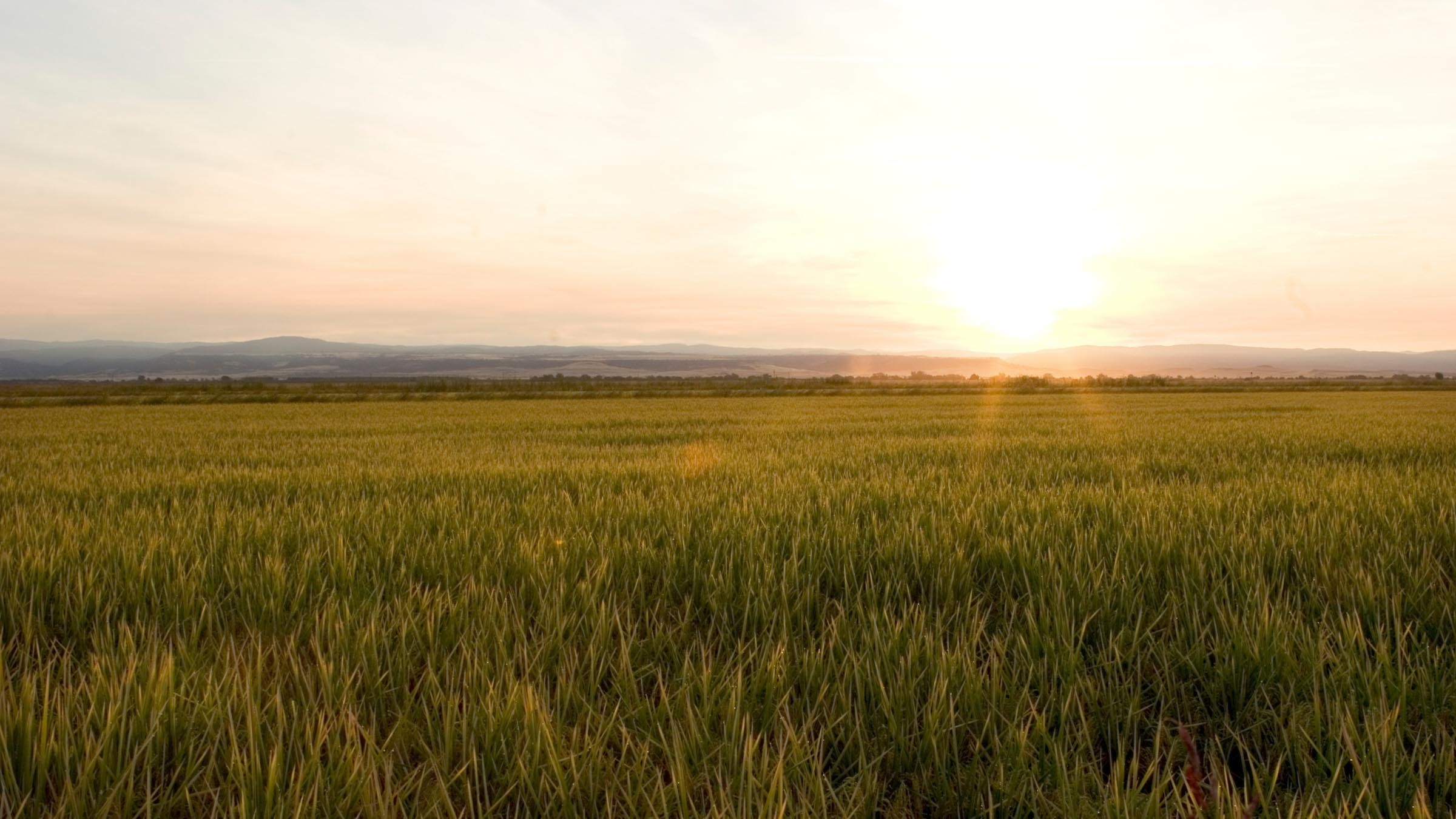This is a photo of a vast, open grassland that extends all the way to the horizon. The scene is illuminated by the sun, which is positioned on the horizon towards the right side of the image, creating a bright, golden-yellow hue that bathes the landscape. The sky, making up the top half of the photograph, is adorned with scattered, illuminated cirrus clouds, suggesting a clear day with no rain. The grassy plain, taking up the lower half of the frame, features tall green grass, with some patches showing signs of browning, possibly indicating the onset of fall. In the distance, beyond the grass, there is a faint, blueish mountain range partially shrouded in a misty, foggy blur. The perspective suggests the photographer is standing in the field, looking outward towards the sun and distant mountains, capturing the serene beauty of this outdoor, nature-filled landscape.